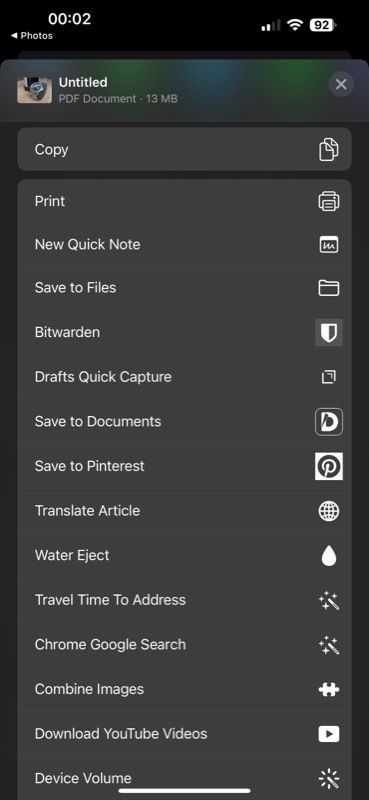This is a detailed screenshot from a smartphone in dark mode, showcasing a context menu. The background is black, and the menu items are listed in white text on the left side, with corresponding icons to the right. Occupying the top row, there's a thumbnail of an image accompanied by the text "Untitled PDF Document, 13 megabytes." In the upper right-hand corner of this row, there is a small, gray circle containing an 'X'.

Underneath, the menu is divided into several options organized in rows. The topmost menu item, enclosed within a rectangular highlight, is labeled "Copy." Below this rectangle, the following options are listed in order: Print, New Quick Note, Save to Files, Bit Warden, Drafts Quick Capture, Save to Documents, Save to Pinterest, Translate Article, Water Eject, Travel Time to Address, Chrome Google Search, Combine Images, Download YouTube Videos, and Device Volume. Each option is paired with a small icon on its right side, uniformly displayed in white.